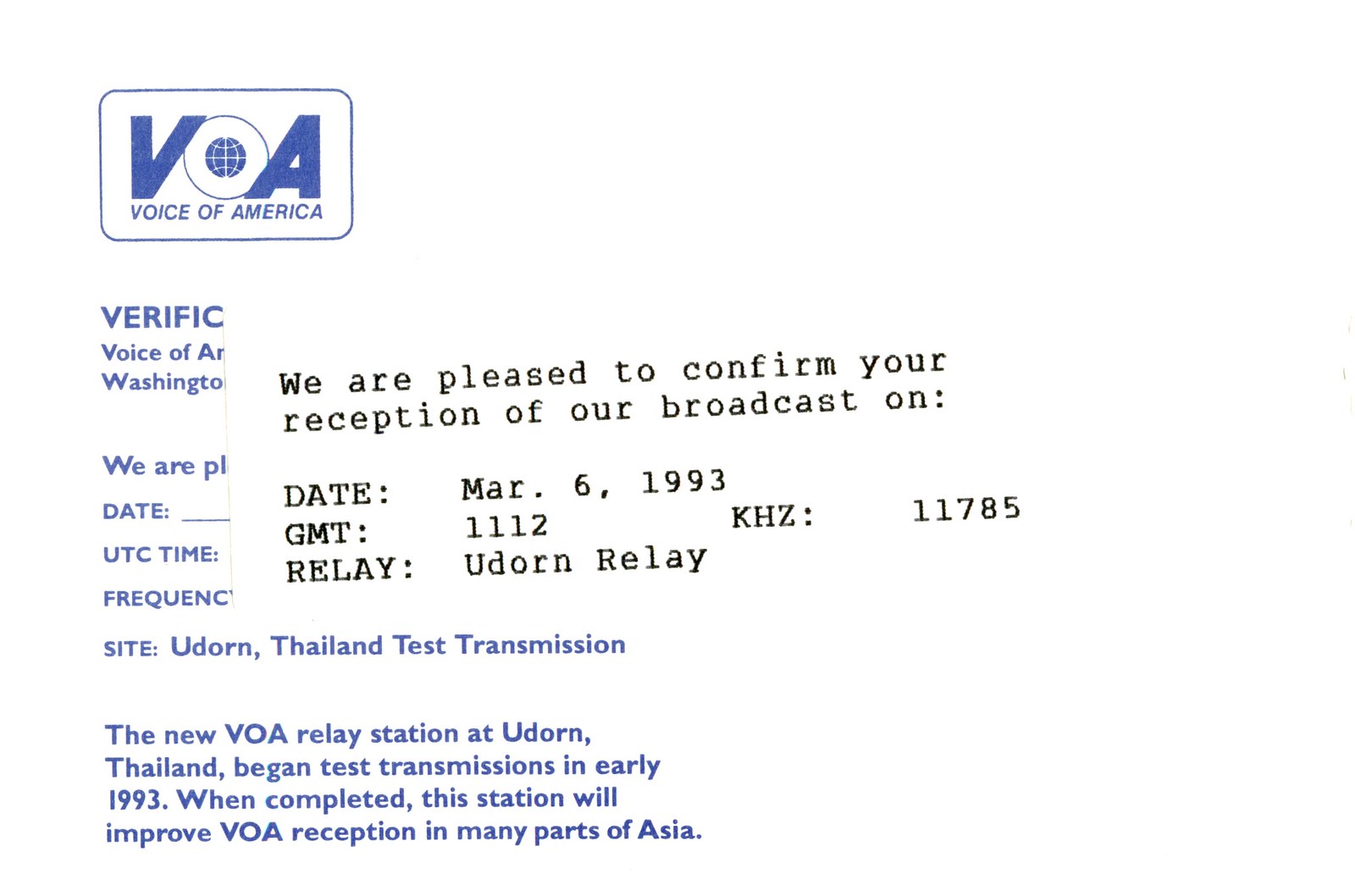The image depicts a telegram-style verification notice set against a plain white background, with the prominent feature being a blue square and the VOA (Voice of America) logo at the top left corner. Inside the 'O' of the VOA logo is a globe, resembling a basketball with section lines. Below the logo, the text reads "Voice of America." The main body of the notice states: "We are pleased to confirm your reception of our broadcast on March 6, 1993, GMT 1-2 kHz 11785 Relay Udorn." Below this, it reads "Site: Udorn, Thailand. Test transmission: The new VOA relay station at Udorn, Thailand began test transmissions in early 1993. When completed, this station will improve VOA reception in many parts of Asia." There appears to be a sticker overlaying some portion of this text, reiterating the confirmation of the broadcast details.